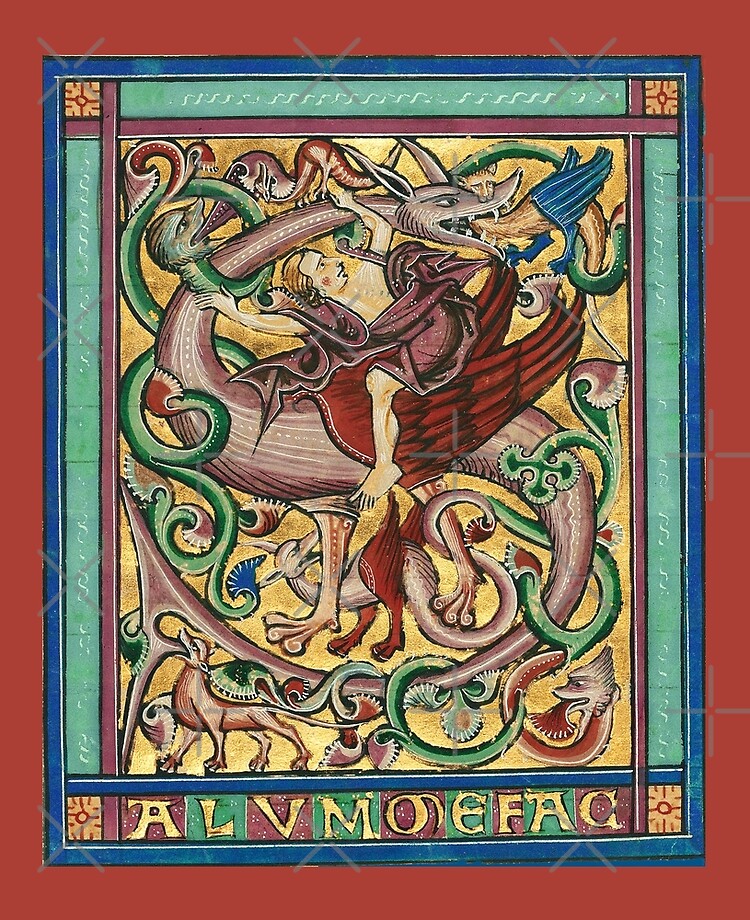This detailed image, styled as an illuminated manuscript from the Middle Ages, is framed by multiple intricate borders: a red outer frame, followed by royal blue, light green, and a purplish color. Inside the additional inner borders—a white border, a black one, a teal patterned border, and another sequence of black, red, white, and black—lies the main scene encased in a blue and aqua frame. The background is enriched with a gold wash, enhancing the vivid depiction within.

Dominating the scene is a mythical chimera-like dragon of mauve and green hues, adorned with long donkey-like ears, a dragon's face, sharp teeth, red wings, and uniquely shaped feet resembling a chicken's. Its body, covered in bizarre, fanciful features, ends in a forked tail. One of the dragon's intriguing traits is its ability to entangle other mythical creatures—each a blend of different animals—in its lengthy, serpentine form. One such creature, peering from the dragon's mouth, resembles a phoenix.

A man, seemingly undisturbed by the chaos, rides atop the dragon's back and grips one of its wings. Among the menagerie around him are a semi-griffin, an animal with a monkey-like face and tentacle-like body, and various other chimeras, including a bird, a green snake-like creature, and deer-like animals with wings.

At the bottom of the image, a set of letters spells A L V M, followed by a glyph resembling an 'O' with an upper ponytail-like flourish, then E, and possibly F A C. The complexity of the text and the mythological imagery together weave a visually stunning tapestry of medieval artistic imagination.